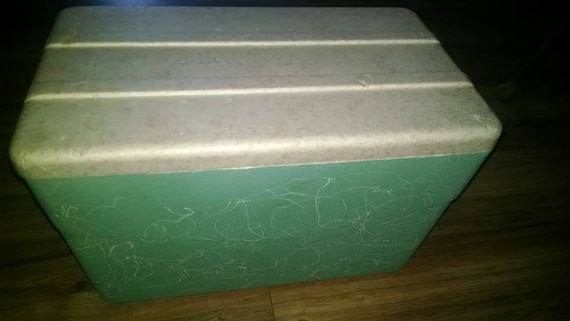The image displays a well-used styrofoam ice chest resting on a wooden floor. The body of the cooler is a light green or aquamarine teal color, heavily marred with random white scratch marks and rounded patterns, indicating frequent use. The top of the cooler is a light gray or white styrofoam lid, designed with smooth, rounded edges. The lid is sectioned into three similarly-sized rectangles divided by horizontal lines. Although the image is grainy and somewhat dark, particularly towards the back where it almost turns pitch black, there is a faint light illuminating the front of the cooler. This reveals a light brown, wooden floor with visible plank separations at the bottom center of the image, where shadows partially obscure the details.